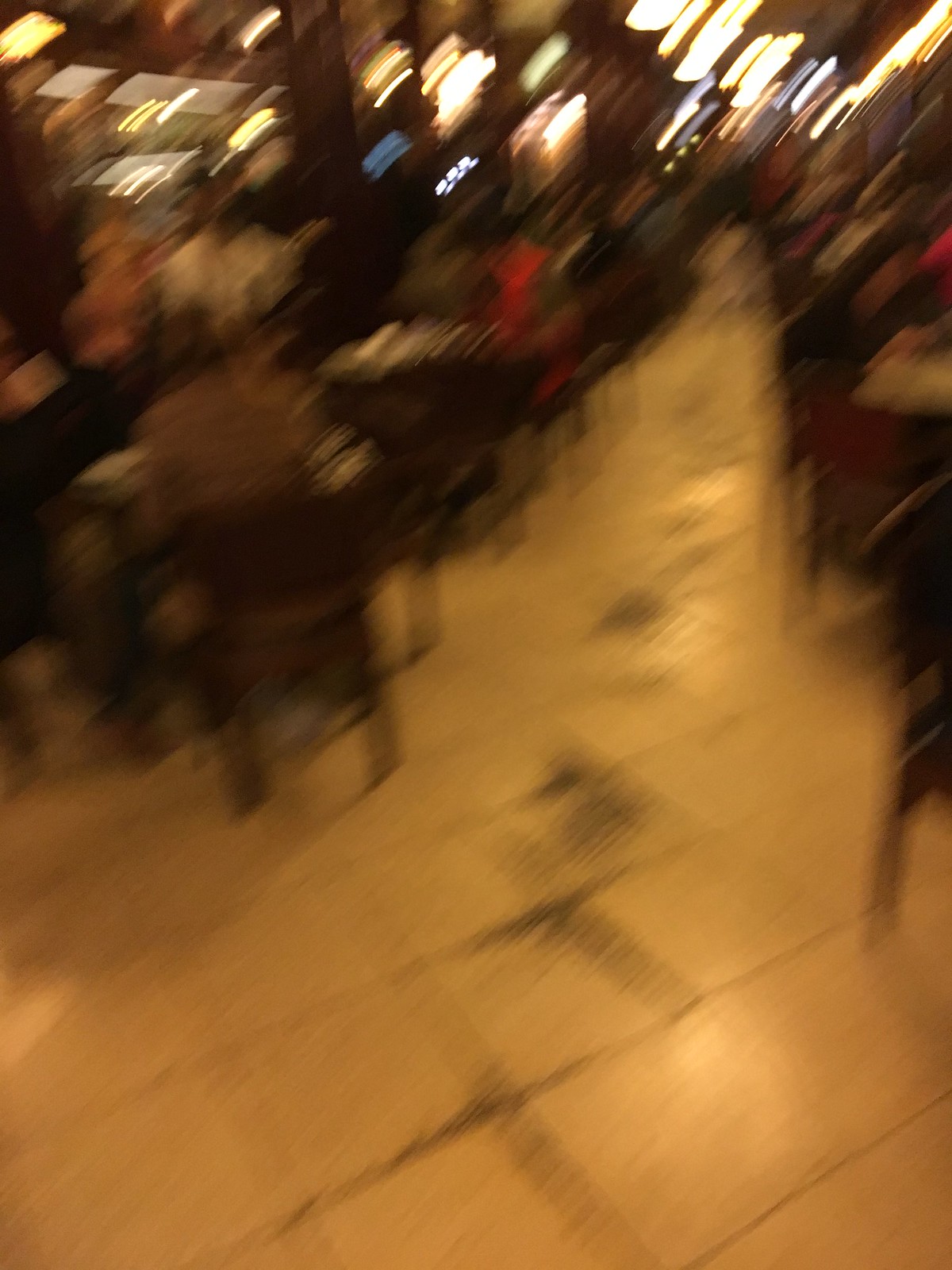This is an extremely blurry photo taken inside what appears to be a busy restaurant. The image, likely captured with a moving smartphone camera, shows a tiled floor that could be either beige or burnt yellow, organized into squares. The floor creates a central path through the scene, lined with tables on both sides. On the left side of the photo, patrons are seated at tables with utensils, while on the right-hand side, a chair concludes the line of tables. The chairs are dark with thin legs and have people, whose faces and bodies are hard to distinguish, sitting in them. Notably, one man wearing tan is visible, sitting with his back to the camera on the left side. The restaurant is illuminated from above, with light reflecting off the tile floor, adding to the overall sense of a bustling dining space.